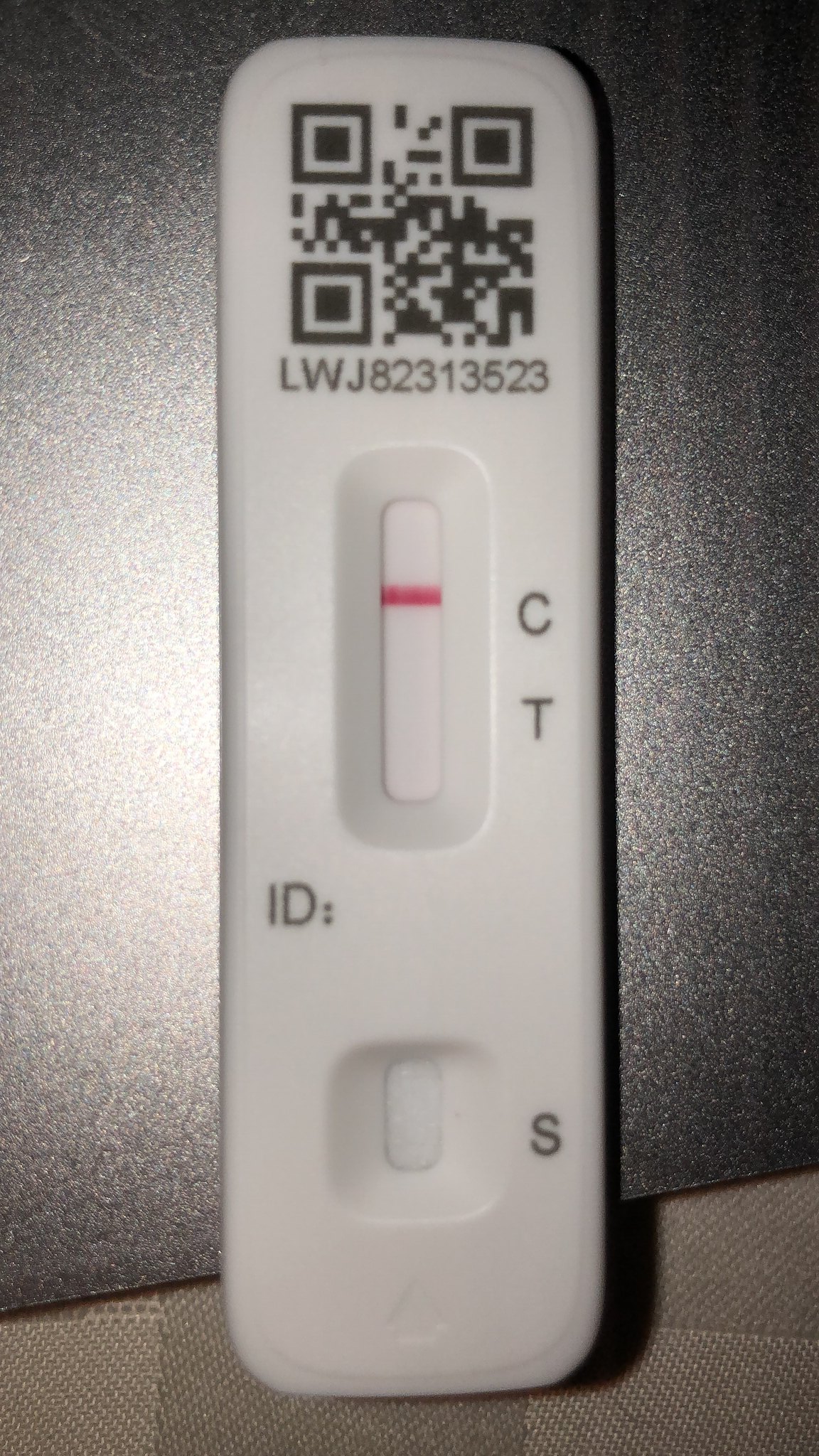In this close-up image, a vertical COVID-19 test is prominently displayed. The test is placed on a two-tone tan surface, featuring a darker tan base that resembles the texture of canvas bins. This surface is characterized by two layers of fabric, one with a horizontal weave and the other with a vertical weave, each with slightly different shades of tan. The backdrop of the image shows a black speckled countertop, which appears darker on the right side due to light reflection.

The COVID-19 test itself has distinctive features. At the bottom, there is an indented arrow pointing upwards towards a concave area marked with an "S." Above this section is black lettering that reads "ID:" on the left side. Moving upwards, another concave portion contains a horizontal red line aligned with a "C." Directly below the "C" is a "T" without any corresponding line. At the top of the test card, a QR code is visible, accompanied by the text "LWJ 823 135 23" underneath it.